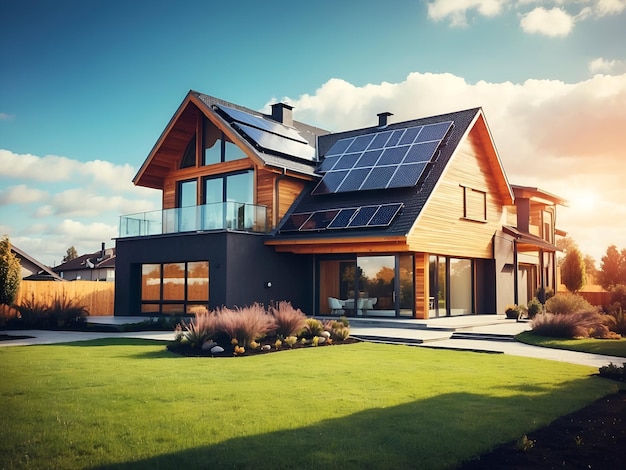This detailed digital rendering captures a modern, elegant two-story house with a pine-colored horizontal wood panel exterior. The house features expansive glass windows on the bottom floor, allowing clear views into the interior, and a large glass balcony on the upper level with a triangular, slanted roof adorned with solar panels. The right side of the house includes a black-painted garage with matching large archway-shaped windows. Surrounding the house is a well-manicured, lush green yard, highlighted by mounds of dirt with various types of bushes and plants in vibrant purple, green, yellow, and brown tones. A gray sidewalk walkway gracefully winds through the yard and up the side of the house. In the background, neighboring houses peek through, enhancing the suburban neighborhood ambiance. The sky is a bright, sunlit blue with scattered white clouds, adding to the overall serene and picturesque setting.